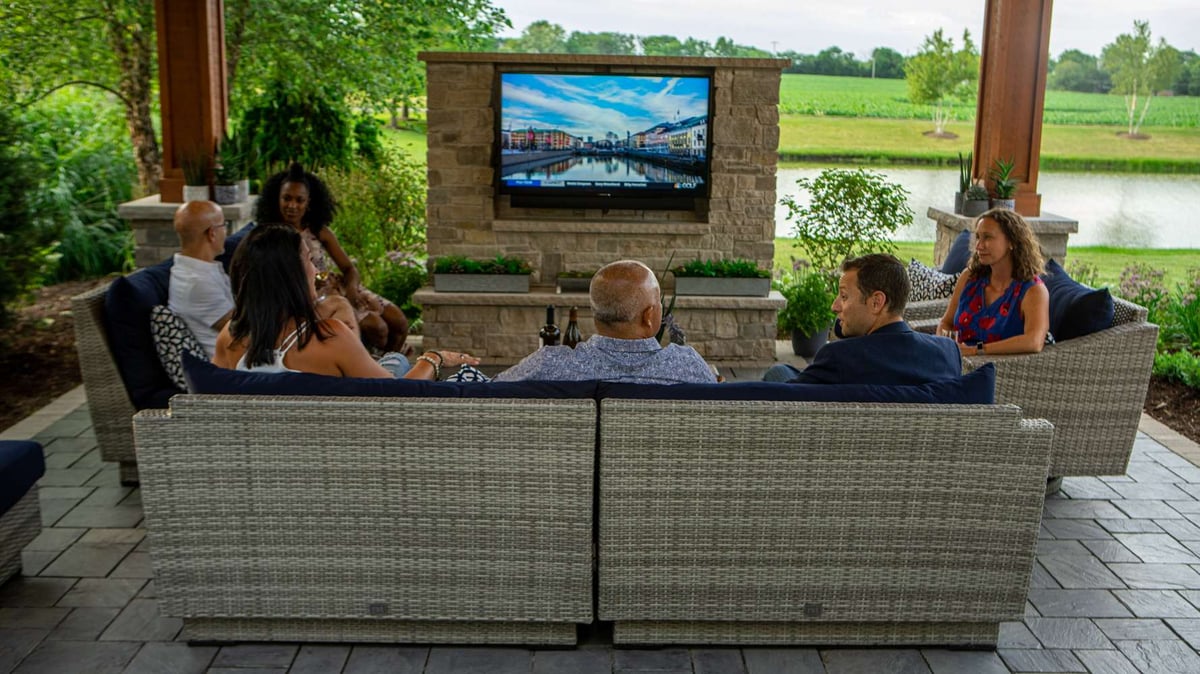The photo depicts a group of six people relaxing on a stylish outdoor patio. The seating arrangement consists of one large rattan-patterned couch with dark blue cushions and two matching love seats positioned perpendicularly on either side. The largest couch, centrally located, hosts three individuals: two men and a woman with dark hair. To the right, a single woman sits on a love seat, while another love seat on the left accommodates a couple. Everyone appears to be engrossed in a large TV screen displaying a serene scene of a European city, possibly Copenhagen, set against a tall brick stand or cabinet. The patio floor is paved with cobblestones and surrounded by well-kept garden beds. In the background, green trees, a grassy area, and a creek or pond contribute to the tranquil outdoor setting.